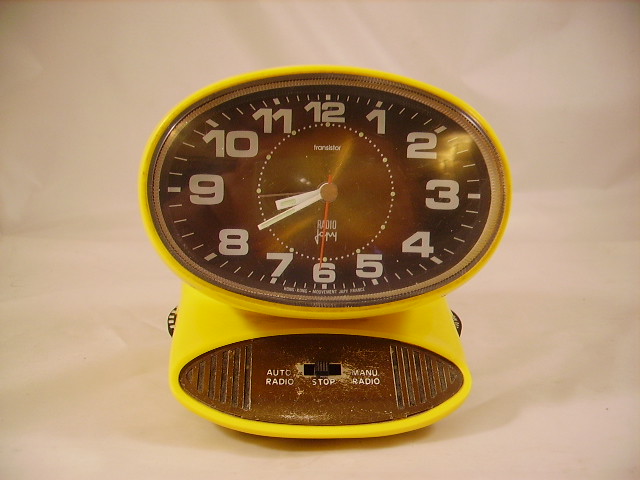In this image, we see a unique, retro-style clock radio set against a tan background, which serves as both the wall behind and the surface on which the device sits. Shadows cast on the background add a touch of dimension, introducing subtle hints of gray. The clock radio itself has a yellow base shaped like a semicircle at the front, which transitions into straight lines towards the back. 

On either side of the device’s front are black dials, positioned on the outer perimeter. At the center of the clock radio is a black oval panel labeled with the words "Auto Radio Stop" and "Manual Radio," featuring a switch in the middle currently set to "Stop." Positioned above this panel is a yellow oval housing a black-faced clock. The clock’s face features the numerals 1 through 12 in white, with hash marks at intervals between each number. The clock reads 8:40, with its hands also appearing in white.